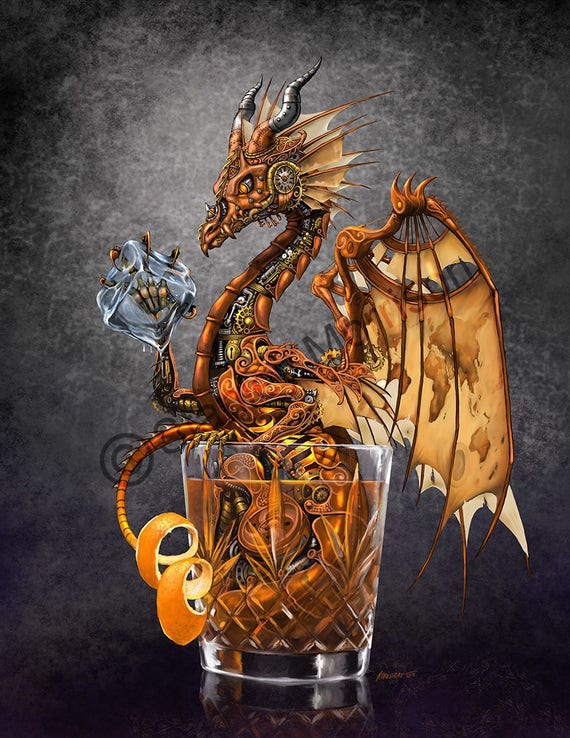The image depicts a fantastical clockwork dragon intricately designed with copper-colored metal parts, nestled inside a clear beveled diamond-patterned cocktail glass. The glass, filled with a brown liquid and wooden pieces, sits against a mottled gray background, lighter in the center and darker at the corners, with a reflective surface below.

The dragon's body, made of interconnected gears and mechanical components, curls inside the glass and extends outwards. Its tail, resembling an orange peel, twists elegantly and curves towards its nose. One of its claws clutches the rim of the glass, while the other, transparent claw holds an ice cube aloft near its face. The dragon's wings, made from parchment-like paper stained brown at the edges, are slightly folded back, supported for flexibility and separation. Its long neck curves sinuously, ending with a pointed beak and two curved horns atop its head.

Sharp claws and horns accentuate the dragon's fierce and intricate design, further emphasizing the blend of fantasy and steampunk elements in its copper, brown, and yellow coloring.